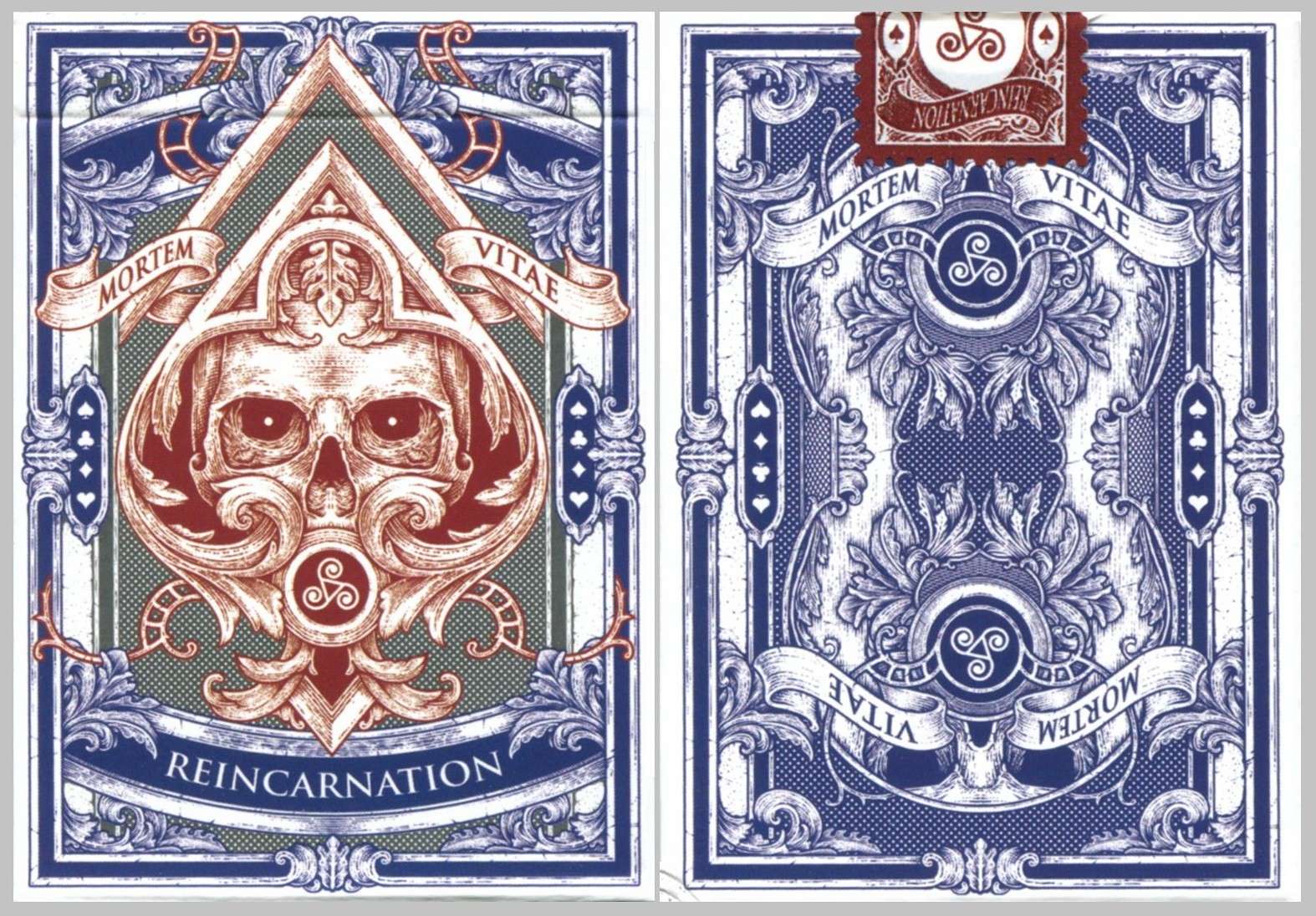The image features two highly detailed and visually striking cards, possibly intended as the front and back of playing cards or as artwork on a deck box. Both cards use a predominantly white background with intricate designs largely rendered in shades of blue.

**Left Card:**
- **Center Region:** Features a green and white checkered pattern with a superimposed, reddish-brown skull. The skull has dotted eyes and is surrounded by a foliage motif in the same reddish-brown color.
- **Mouth Area:** The skull's mouth forms a circle that houses a triangle with three spirals—an intriguing symbol that also appears on the other card.
- **Bottom Banner:** Contains the word "REINCARNATION" and is styled as a red-printed ribbon. Flanking this ribbon are the Latin words "MORTEM" and "VITAE," meaning death and life, respectively.

**Right Card:**
- **Design:** Predominantly blue with a symmetrical floral pattern. 
- **Symbols:** Features the triangular symbol with three spirals at both the top and bottom.
- **Banner:** Like the left card, it displays "MORTEM" and "VITAE" separated by "REINCARNATION," styled in a similar ribbon-like fashion.
- **Seal:** A brown, postage stamp-like seal marked with the word "REINCARNATION" and the triangular symbol adds another layer of detail and suggests authenticity.

The recurring themes of life, death, and reincarnation, alongside the unique triangular symbol, hint at a deeper symbolic context. The detailed symmetrical patterns and recurring iconography imply these cards might be part of a spiritual or mystical tool, possibly used for divination or themed playing cards within a unique, artistically designed deck.